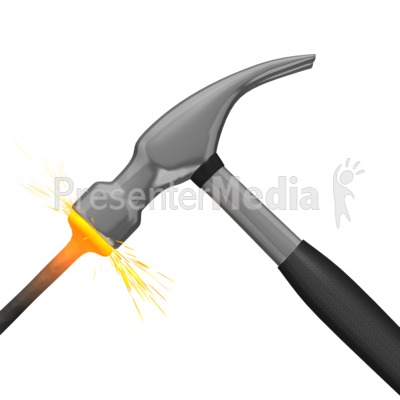The image depicts a strikingly detailed scene of a hammer hitting a nail against a white background. The hammer, positioned on the right side, features a black handle transitioning to silver with a black ring near the head. The head of the hammer is dark gray, with its claw facing the upper right. As the hammer strikes the nail on its left side, a burst of orange sparks erupt from the point of contact. The nail’s tip glows orange, fading to black toward its base. Superimposed on the background, there is gray text reading "Presenter Media," accompanied by an icon of a simplistic human figure. The figure stands with one arm raised, a circle for a face, and three lines above the head, conveying a dynamic, animated pose. The overall aesthetic suggests a stylized representation, likely digital in nature.